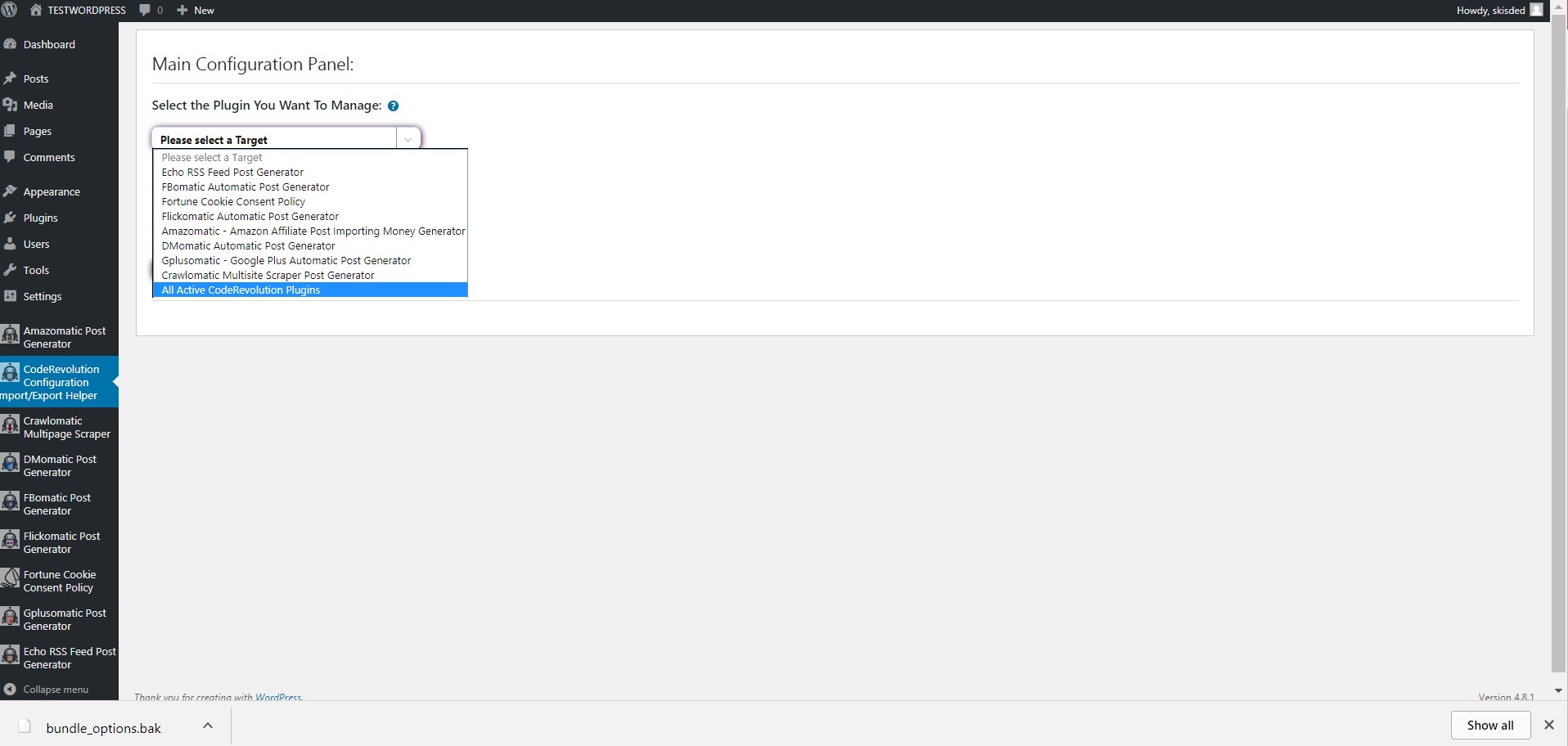The screenshot depicts a WordPress website currently on the 'Main Configuration' page of a plugin management panel. In the upper-left corner, the site is labeled 'Test WordPress.' A navigation bar is present on the left side of the screen, featuring several options: Dashboard, Posts, Media, Pages, Comments, Appearance, Plugins, Users, Tools, Settings, Anamorization at AMAZOMATIC Post Generator, and Code Revolution Configuration. The 'Import Export Helper' is highlighted in blue, indicating that is the active page.

The main section of the page includes a heading that reads "Main Configuration Page," followed by instructions to "Select the plugin you want to manage. Please select target." Below this heading is a list of various post-generating plugins, including ECHORSSV Post Generator, FBMATIC Automatic Post Generator, Fortune Cookie Consent Policy Generator, FLICOMATIC Automatic Post Generator, AMAZONAMATIC Amazon Affiliate Post Importing Money Generator, DEMOMATIC Automatic Post Generator, GLIPSOMATIC Automatic Post Generator, Google Plus Automatic Post Generator, and PROLOMATIC Multi-Site Scraper Post Generator. Each of these plugins is categorized under "All Active Code Revolution Plugins."

The interface features a clean design with a color scheme consisting mainly of blue, black, white, and gray. The background is white, lending a stark contrast to the black text, enhancing readability.